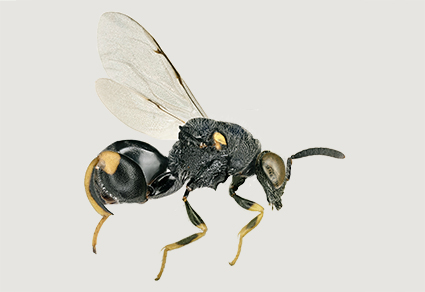This is a detailed side-view, close-up photograph of a hornet against a light gray, off-white background. The hornet, primarily black, features a rough-textured thorax and a large, shiny black abdomen with a prominently displayed long stinger. It has two transparent wings extending from its thorax and positioned up and outwards. The head of the hornet is black, adorned with large golden eyes and black antennae stretching forward. A small yellow spot is present on the thorax near where the wings attach, and another yellow spot marks the rear of the abdomen. The legs, three of which are visible, start black and transition into yellow towards the bottom. The intricate details of the hornet's segmented body and striking coloration are clearly captured in this photograph.